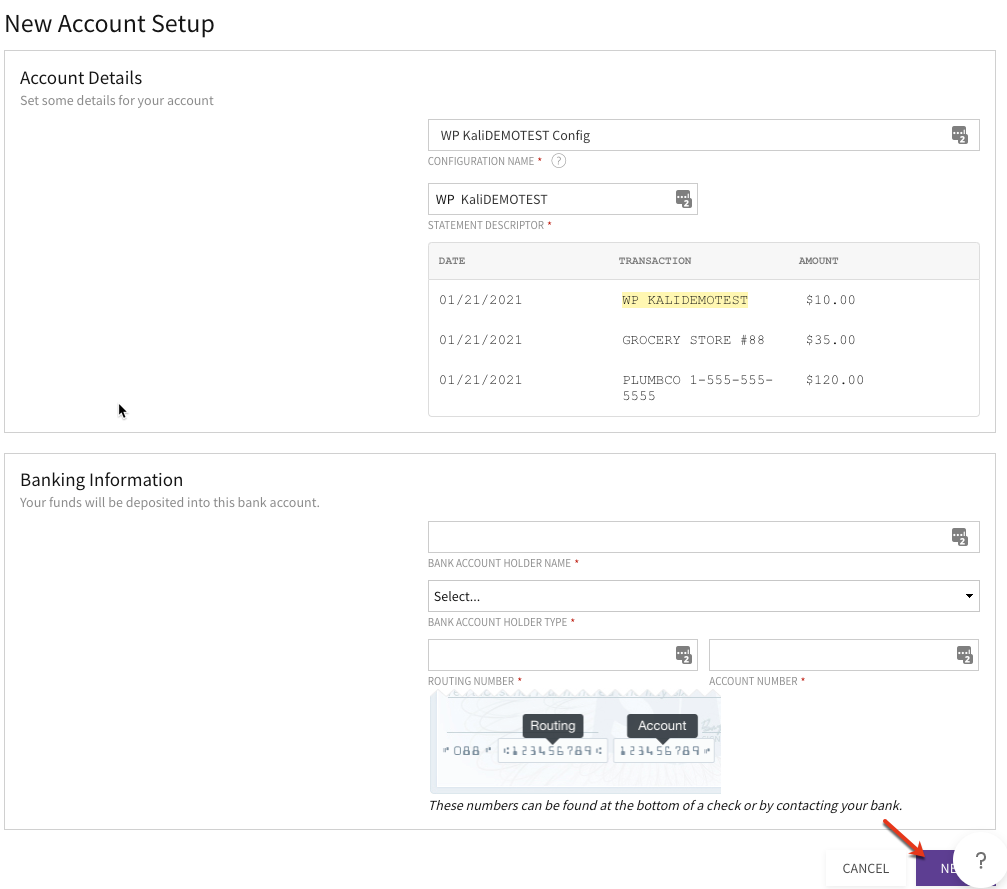The image is a screenshot featuring a clean, solid white background. The central focus is on two light gray-lined boxes, situated one above the other. The lower box commands the viewer's attention first, where prominently in the upper left corner, bold text reads "Banking Information." Directly beneath this title, the accompanying text states, "Your funds will be deposited into this bank account."

To the right of this text, a form is neatly arranged. The first field in the form requests the "Bank Account Holder Name." Below this field, there is a dropdown menu labeled "Bank Account Holder Type," currently displaying the default option "Select." Further down, two adjacent fields are available: the left one labeled "Routing Number" and the right one labeled "Account Number."

Beneath these fields, an illustrative image showcases a corner of a check. On this check, the routing number and account number are visibly displayed, providing visual guidance. An informative note beneath the image explains that these numbers can be found at the bottom of a check or by contacting your bank for assistance.